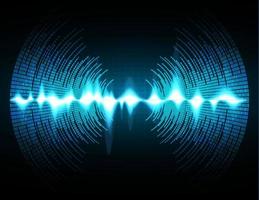The image is a vibrant digital graphic dominated by shades of blue and black, projecting a futuristic and abstract aesthetic. At its core is a central line of bright blue light with varying heights, resembling an audio waveform or equalizer readout, transitioning to white at the peaks. Surrounding this pulsating light is a circular pattern of lines radiating from the center, which evoke the organized, sweeping movements of a radar display but do not explicitly depict one. The black background accentuates the brightness of the blue and white elements, giving them a glowing, almost ethereal quality. On the left and right sides, box-like structures form lines that appear to create a broken tunnel effect, interrupted at the top and bottom. The luminescent, wavy frequency spikes and circular motifs contribute to a dynamic and intriguing visual, suggesting themes of technology and music, perfect for web or logo design, though the graphic itself remains text-free.